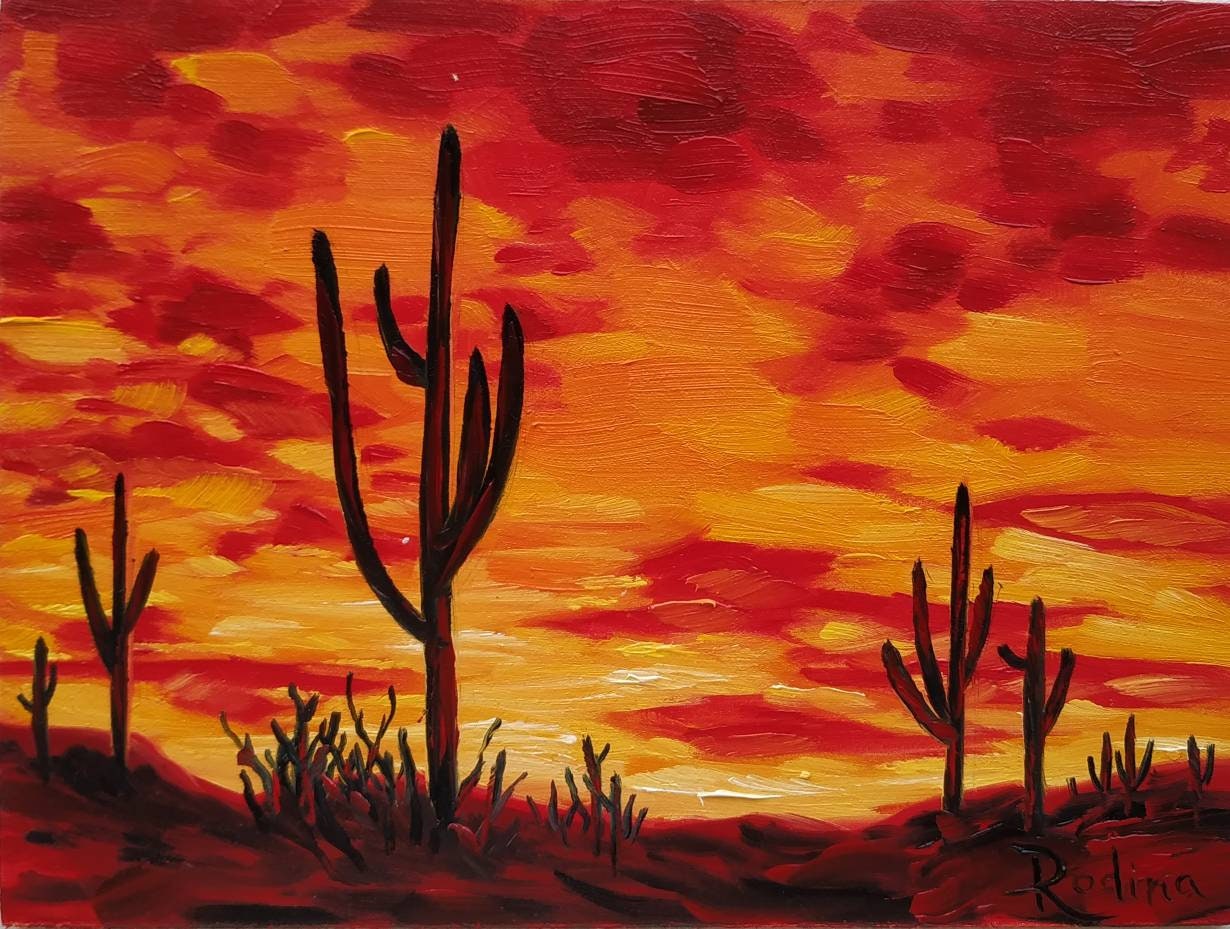This vibrant painting, signed by the artist Rodina in the bottom right corner, captures a dramatic desert landscape at sunset. Dominated by a fiery sky, the image features sweeping streaks of red, orange, and yellow, with hints of pink and white near the horizon. Covering roughly 80% of the canvas, the sky transitions from yellow at the bottom to deep red at the very top, creating an intense and vivid backdrop. The desert ground is a striking shade of red, possibly symbolizing the extreme heat, and is dotted with cacti that are meticulously outlined in black and dark red. The largest cactus is positioned to the left, surrounded by numerous smaller ones and additional desert flora. In the distant background, subtle mountains add depth to the landscape, enhancing the sense of vastness and isolation in this striking and intense portrayal of a desert at sunset.